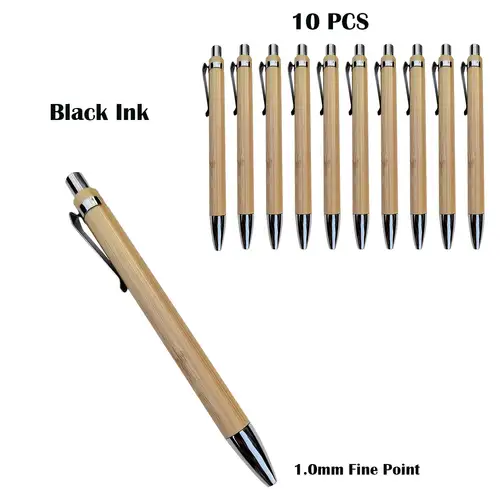This image features a collection of ten identical ballpoint pens arranged side by side against a plain white background. At the top of the image, in bold black text, it reads "10 PCS," indicating the quantity. To the left, it states "black ink" in thick black letters. These pens have a beige or creamy brown body that gives a faux wood appearance. Each pen is equipped with a silver tip and a matching silver clicker at the top for retracting and extending the ink point. They also have a silver metal clip on the side for attaching to pockets. An additional pen is shown angled with the tip toward the bottom right corner of the image and the clip facing the left side, mirroring the alignment of all the pens. The bottom right corner indicates the pen's specifications with the text "1.0 mm fine point," highlighting the fineness of the ballpoint tip. None of the pen tips are extended in the image.